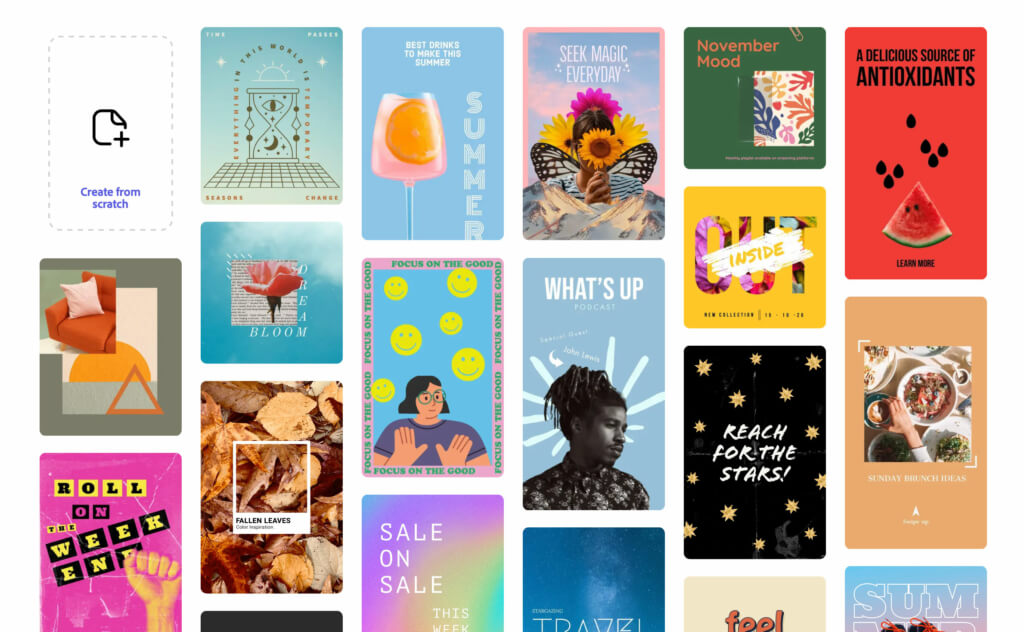The mosaic image is composed of various smaller images arranged within squares, each depicting a unique design. In the upper left corner, a square is bordered with dotted lines and the text "Create from scratch," suggesting a tutorial-like layout for creating the designs. The top row begins with an hourglass timer featuring a moon and an eyeball in the upper section. To its right, a vibrant pink cocktail glass with an orange slice sits alongside the vertically oriented word "Summer." Continuing right, a square adorned with multicolored flowers and butterfly wings contains the motivational phrase "Seek magic every day." Adjacent is a green square labeled "November mood."

The next row adds more visual interest. A delectable watermelon slice with black seeds illustrates "A delicious source of antioxidants." In the center, a blue background features the white text "What's up" and a man with dreadlocks wearing a buttoned collared shirt. Left of this, an animated figure with short black hair and disproportionately large hands is set against six yellow smiley faces. On the far left, a pink square with block-style text spells out "Roll on the weekend."

Each square exudes a distinct vibe, collectively creating a visually engaging and eclectic collage.